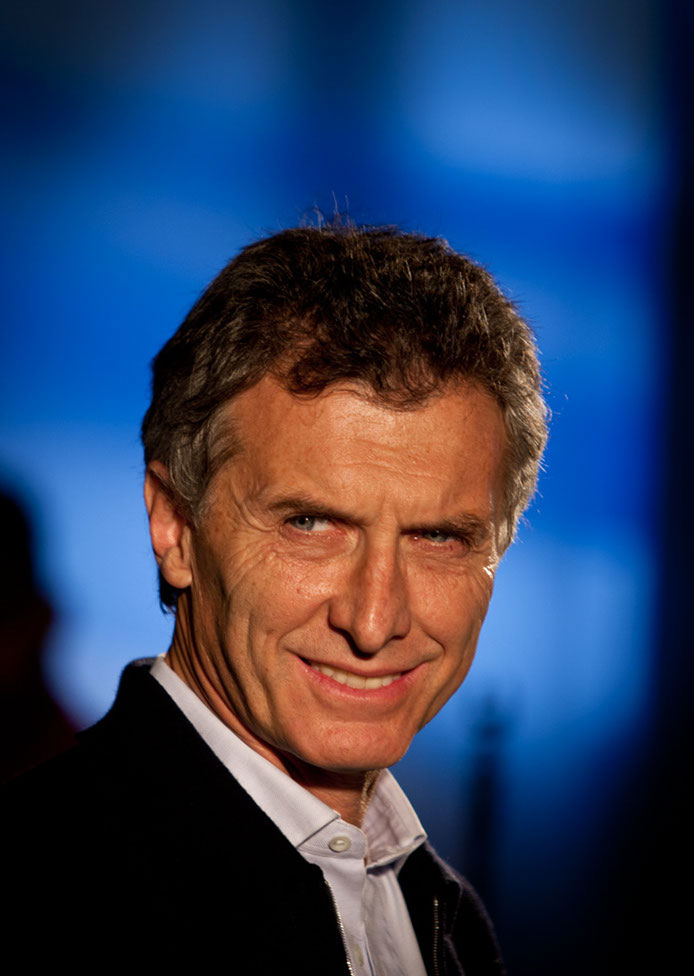The image depicts an older man with a partial smile, revealing his teeth, as he looks to his right with his eyes slightly turned to the left. His curly hair is a mix of brown and slightly gray, and his eyes are either gray or blue, possibly light green and silverish. He has noticeable crow’s feet around his eyes. He is dressed in a black zip-up jacket or sweatshirt, paired with a white collared shirt featuring clear buttons. The background of the photo is an ocean blue color with varying shades of blue and black, especially around the edges, creating a visual blur that isolates the man's face and upper body.